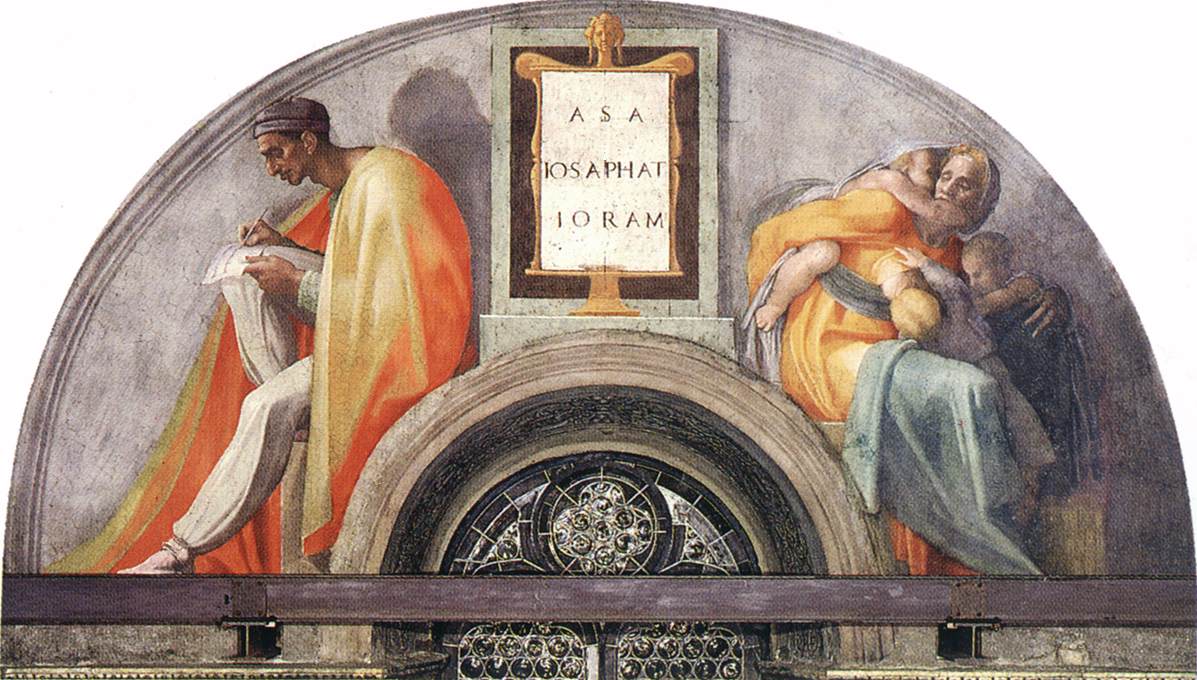The mural, displayed prominently on the entrance of a church, is a stunning semi-circular painting with a detailed composition. The background is a cold blue-gray, accentuating the figures in the foreground. On the left, a man adorned in a gold cloak over white trousers and white shoes is intently writing on a white piece of paper, his head bowed in concentration. He wears an orange cape and a hat, adding to the vibrant color palette. On the right, a woman dressed in an orange robe with white cloth accents cradles three children who cling to her for refuge—one on her back and two near her knees. She gazes towards the man. Both figures are elegantly depicted with intricate details that highlight their roles and attire. The center of the mural features a white scroll with the names "Asa, Josaphat, and Joram" inscribed, framed by the imagery of the figures. The church door itself, visible at the top of the mural, appears elaborate, almost as if adorned with jewels or silver leaf, enhancing the mural's majestic presence.